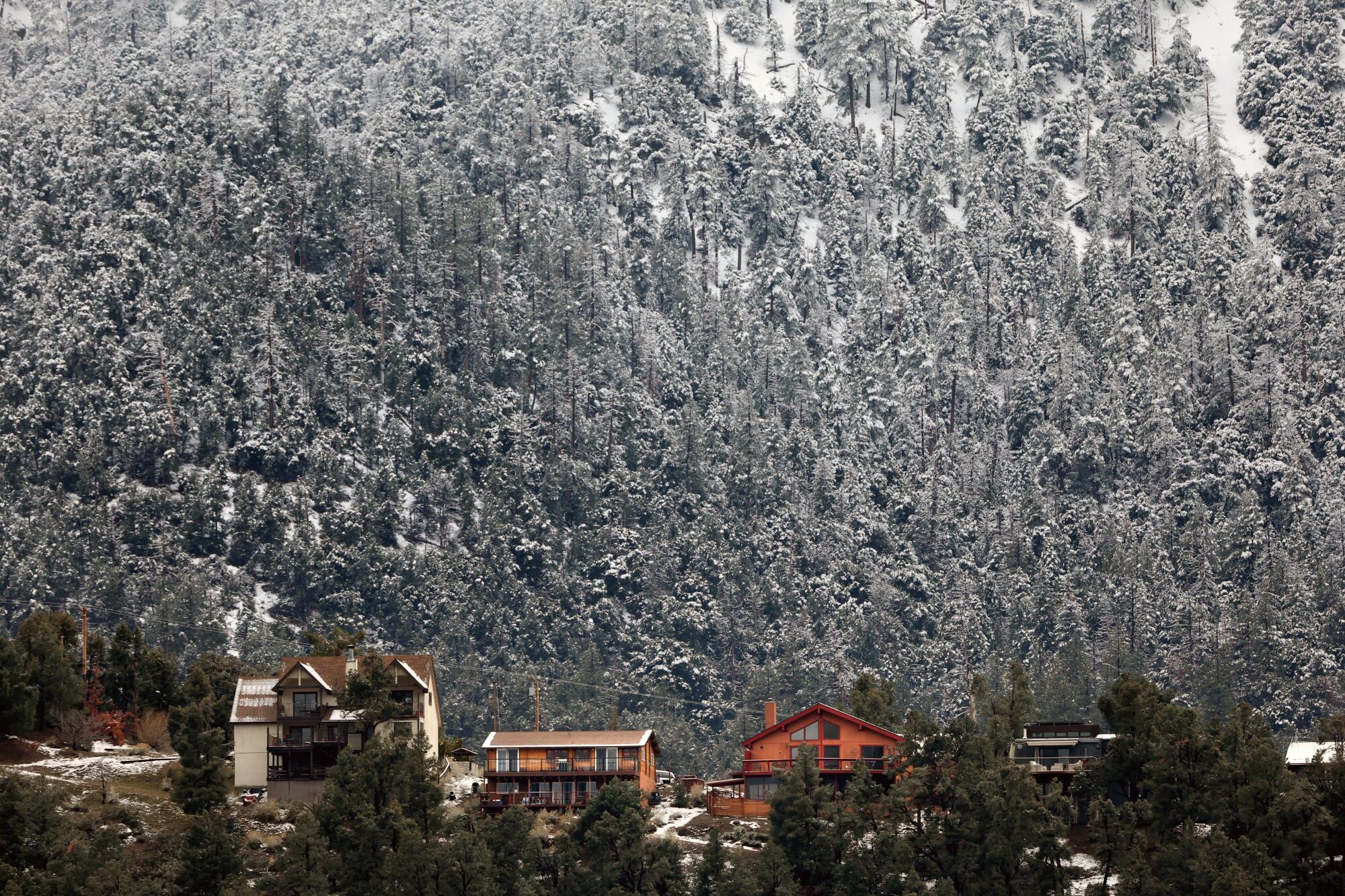The photograph captures a picturesque wintry scene of a mountain or hillside densely populated with trees blanketed in snow. The majority of the image is dominated by these snow-covered trees, creating a wall of white, dusted foliage. Amidst this frosty landscape, the ground scarcely peeks through the thick forest. At a lower elevation, nestled at the bottom of the image, there are about five distinct houses, possibly cabins, in close proximity to each other. These houses vary in color—there's a white and brown house, an orange one, a red-orange one, and another with a modern black and white design. The area around these houses features trees that remain green and snow-free, suggesting either a lower elevation or that the snow has been cleared. This charming contrast between the snowy upper slopes and the more temperate lower area hints at the diverse microclimates of this idyllic winter retreat.